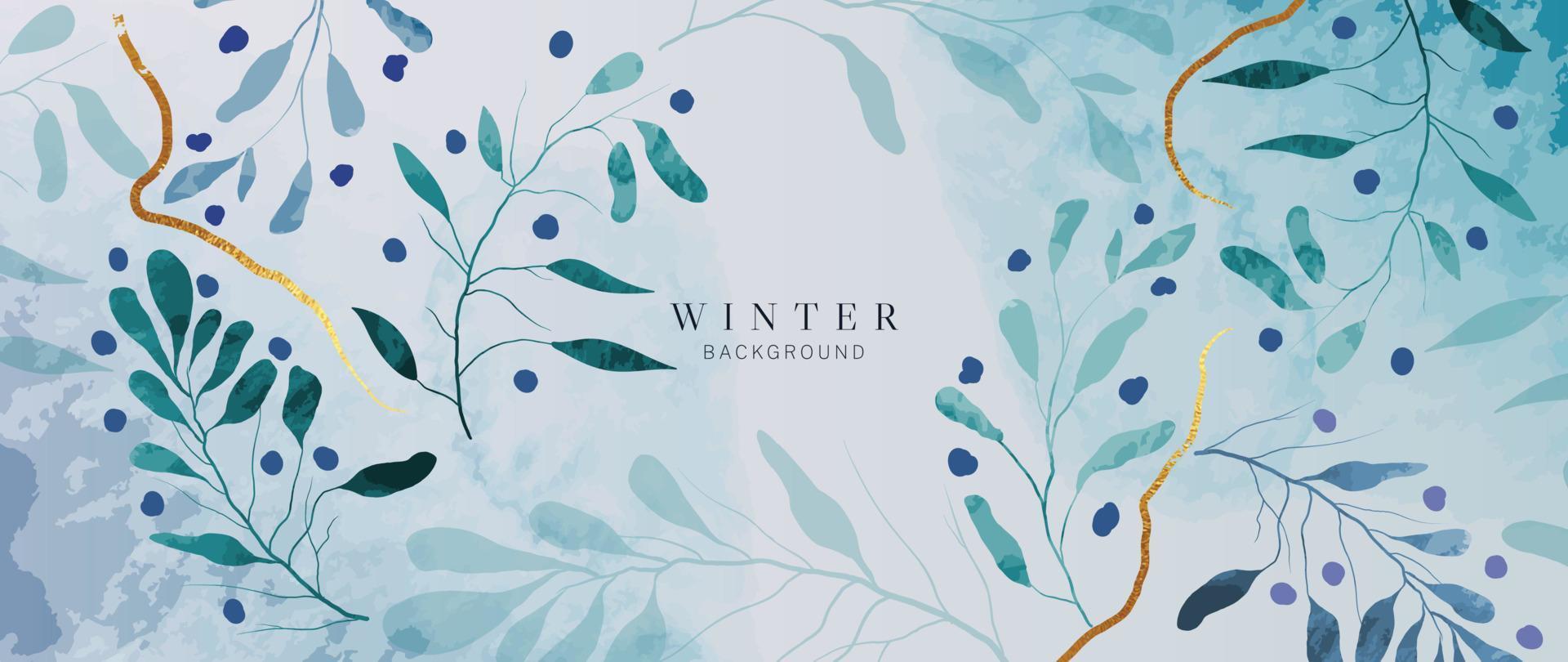The image appears to be an advertisement for a desktop background, featuring a winter theme prominently displayed at its center. The text "WINTER BACKGROUND" is written in black, with "WINTER" in bold, capital letters above a smaller, non-bold "BACKGROUND". This text stands out against a visually striking, wide canvas.

The artwork itself resembles a watercolor painting or a digital creation, composed of branches and leaves in various shades of light greens, blues, off-white, teal, and grays. The delicate twigs and stems seem to emerge and swirl around the canvas, with leaves positioned at their ends. Additionally, the branches host little blue circles and gold foil-like strings, creating an intricate, whimsical pattern. The background gradients from an off-white center to teal at the top right and bluish tones at the bottom left, lending a harmonious blend of wintry colors and elements to the overall composition.